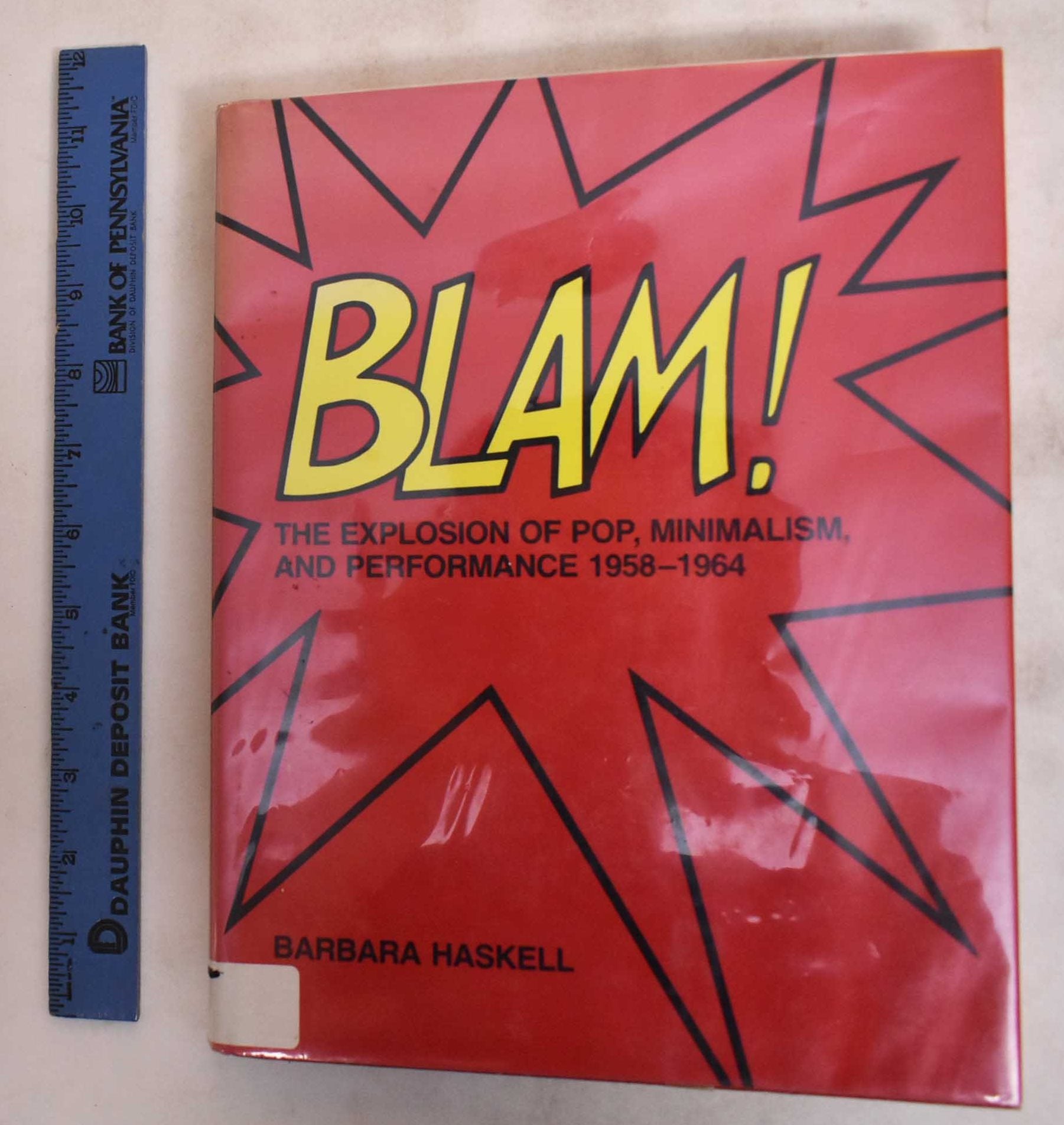The image shows a book with a glossy hard cover sitting on a white table. The book, approximately one foot tall as indicated by a blue ruler marked with "Dauphin Deposit Bank, Bank of Pennsylvania" placed vertically next to it on the left, features a predominantly red background. At the center of the cover, a dramatic comic-style explosion graphic, composed of straight lines forming a series of triangles without hypotenuses, frames the bold yellow text "BLAM!" with a black outline. Beneath this, in black text, the subtitle reads "The Explosion of Pop Minimalism and Performance, 1958-1964." The author's name, Barbara Haskell, is positioned in the lower right corner, while a small white sticker is visible in the lower left corner of the cover.